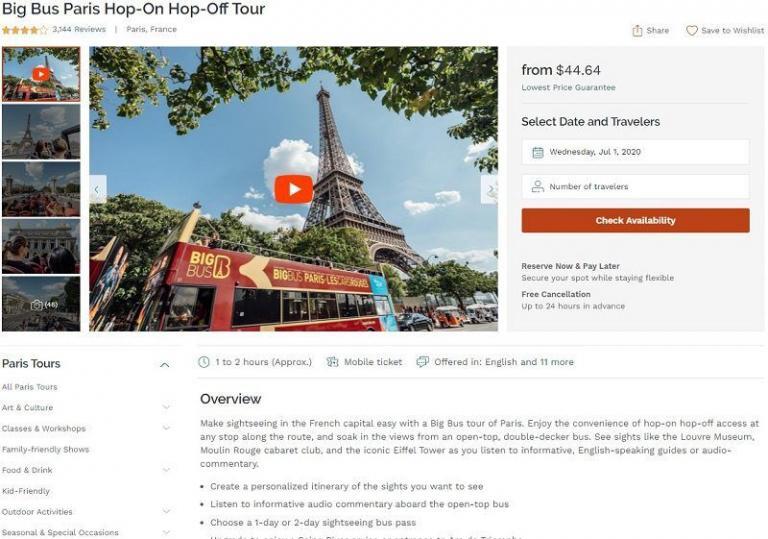**Detailed Caption:**

This is a vibrant color screenshot from an unspecified web page promoting the "Big Bus Paris Hop-On Hop-Off Tour". At the top, the banner proudly displays an average rating of four stars out of five, based on 3,144 reviews, and highlights Paris, France as the location. 

The primary image features a stunning photograph of the Eiffel Tower set against a vivid blue sky adorned with fluffy white clouds. The corners of the photo capture the tops of nearby trees, adding to the picturesque scene. Dominating the center of the picture is a striking red double-decker bus emblazoned with "Big Bus" in gold lettering.

Beneath the image, pricing details indicate that tours start from $44.64 with a lowest price guarantee. Users are prompted to select the date and number of travelers for their tour, providing an example date of Wednesday, July 1st, 2020. The page encourages users to check availability and offers the option to reserve now and pay later. It also highlights the flexibility of securing a spot with free cancellation up to 24 hours in advance.

At the bottom left corner, there is a list of categories linked to the tour, including "Paris Tours", "All Paris Tours", "Art and Culture", "Classes and Workshops", "Family-Friendly Shows", "Food and Drink", "Kid-Friendly", "Outdoor Activities", and "Seasonal and Special Occasions". The tour duration is approximately one to two hours and offers a mobile ticket redeemable in English and 11 other languages.

The overview emphasizes the ease of sightseeing in Paris with the Big Bus Tour, highlighting the convenience of Hop-On Hop-Off access at any stop along the route. It invites travelers to enjoy the view from an open-top double-decker bus whilst visiting iconic landmarks such as the Louvre Museum, the Moulin Rouge Cabaret Club, and the Eiffel Tower. The tour also includes informative commentary delivered by English-speaking guides or via audio recordings. Visitors can tailor their itinerary to their interests and choose between a one-day or two-day sightseeing bus pass for maximum flexibility.